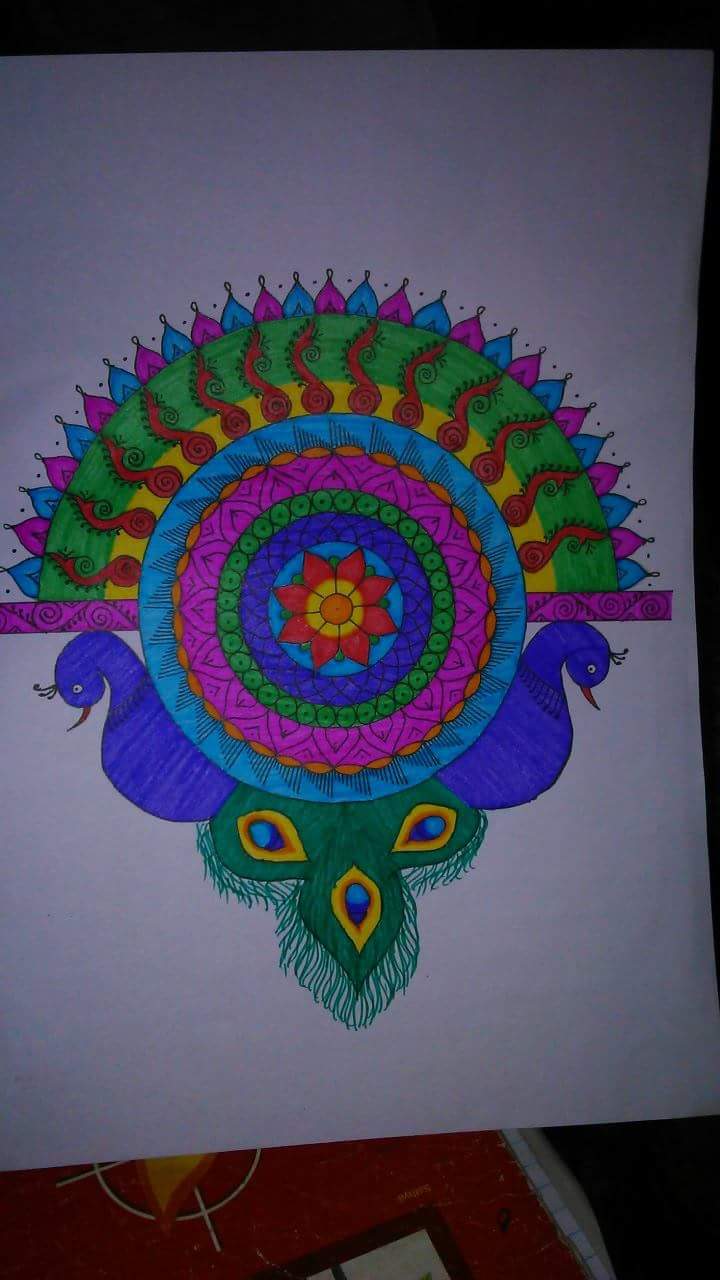The drawing depicts two vividly colored peacocks on white paper. Their tails elegantly merge in the center of the artwork to form an intricate eight-petal flower, with an eye-catching orange circle at its core. The petals radiate in vibrant red, surrounded by concentric rings of alternating colors: light blue, dark blue, green, hot pink, and medium blue. A horizontal line bisects the image, adding a visual anchor for the composition. Above this line, the fan-shaped tail feathers showcase an alternating pattern of pink and blue hues. Green and yellow semicircular sections, adorned with red markings, provide additional layers of complexity. The blue peacock heads face away from each other, positioned on either side of the outer blue ring that encircles the central flower. Beneath this, their bodies extend downward, culminating in an elaborate tail with a three-eyed feather motif.